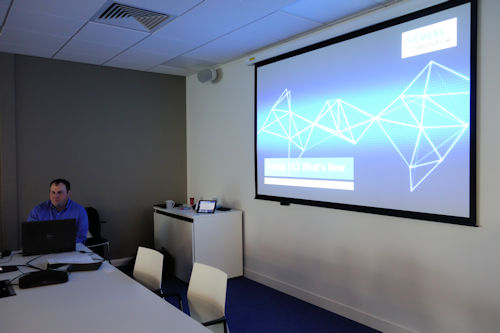The image is a horizontal color photograph capturing a detailed indoor office scene. The ceiling comprises white square tiles, featuring a prominent vent at its center. The back wall is dark gray, while the side wall is off-white, topped with a white baseboard at the floor junction. Foregrounding the office setting, at the lower-left quadrant, a man with black hair sporting a blue shirt is seated in front of a black laptop, which is placed on a long white table. Surrounding him are assorted papers and black objects, along with some visible black wiring and boxes on the table.

Adjacent to the man are two cream-colored modern chairs with black armrests. To his right, a cream-colored filing cabinet is positioned, adorned with a white cup on the left and a small square monitor on the right. In the background, a large screen with black outlines occupies the back wall, displaying a blue, green, and aqua abstract design dominated by white triangular shapes and three noticeable banners. The floor of the room is covered in dark blue carpeting, enhancing the professional atmosphere. The shadow cast by the desk and chairs creates a subtle contrast at the base of the walls, adding depth to the overall scene.